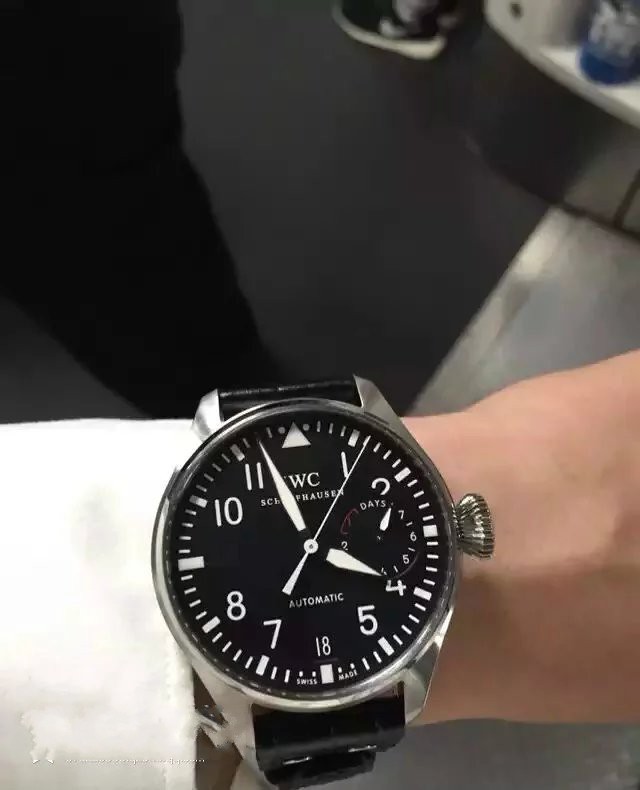This detailed close-up photograph captures a men's wristwatch on a Caucasian person's left wrist, adorned with a long-sleeved white cotton shirt. The watch features a sophisticated black face with white numerals and hands, including a smaller sub-dial for days around the right middle. The time displayed is between 3:56 and 4:56. The watch’s bezel and band attachments are made of silver or white gold, offering a sharp contrast against the predominantly black, potentially leather or two-toned wristband. The silver-trimmed face stands out with distinct detailing: a white triangle at 12 o'clock, white lines at 3, 6, and 9 o'clock, and more traditional numerals at other positions. The background is blurred, revealing partial details such as grey flooring, a small shelf, a hint of a black floor, and the blurred outline of black Nike shoes.